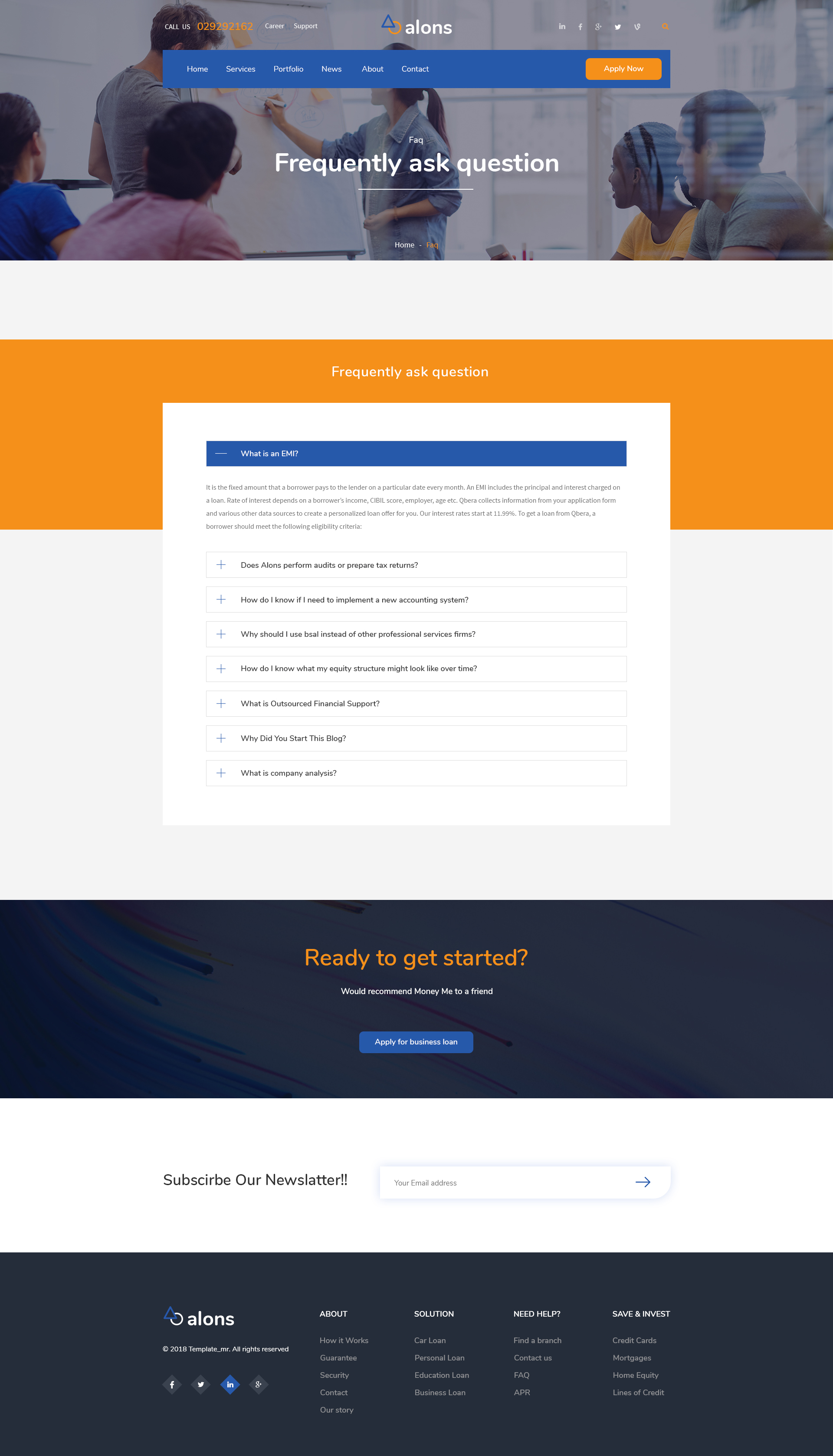The screenshot depicts the homepage of the website "Allons" (spelled A-L-L-O-N-S). The website's logo, positioned at the top, is a unique combination of an interconnected triangle and square. The header includes tabs for various social media platforms, with visible icons for Facebook and Twitter, and additional menu options such as "Home," among others that are partially obscured.

The main content of the page features a photograph capturing a conference room scene with six individuals. The group consists of three women and three men. One woman and one man are standing, engaged in an active discussion as the woman writes on a large board, with the man positioned on the opposite side. The remaining four team members are seated, attentively observing the interaction.

Below the image, a section labeled "Frequently Asked Questions" is present, though obscured by a white box, rendering the text unreadable. Further down the page, a prominent banner invites users to "Get Started," accompanied by what appears to be an "Apply Now" button.

Subsequently, there is a section encouraging visitors to "Subscribe to our Newsletter." The footer area mirrors the social media and logo display from the header, alongside additional navigation links such as "About," "Solutions," "Need Help," and "Save and Invest."